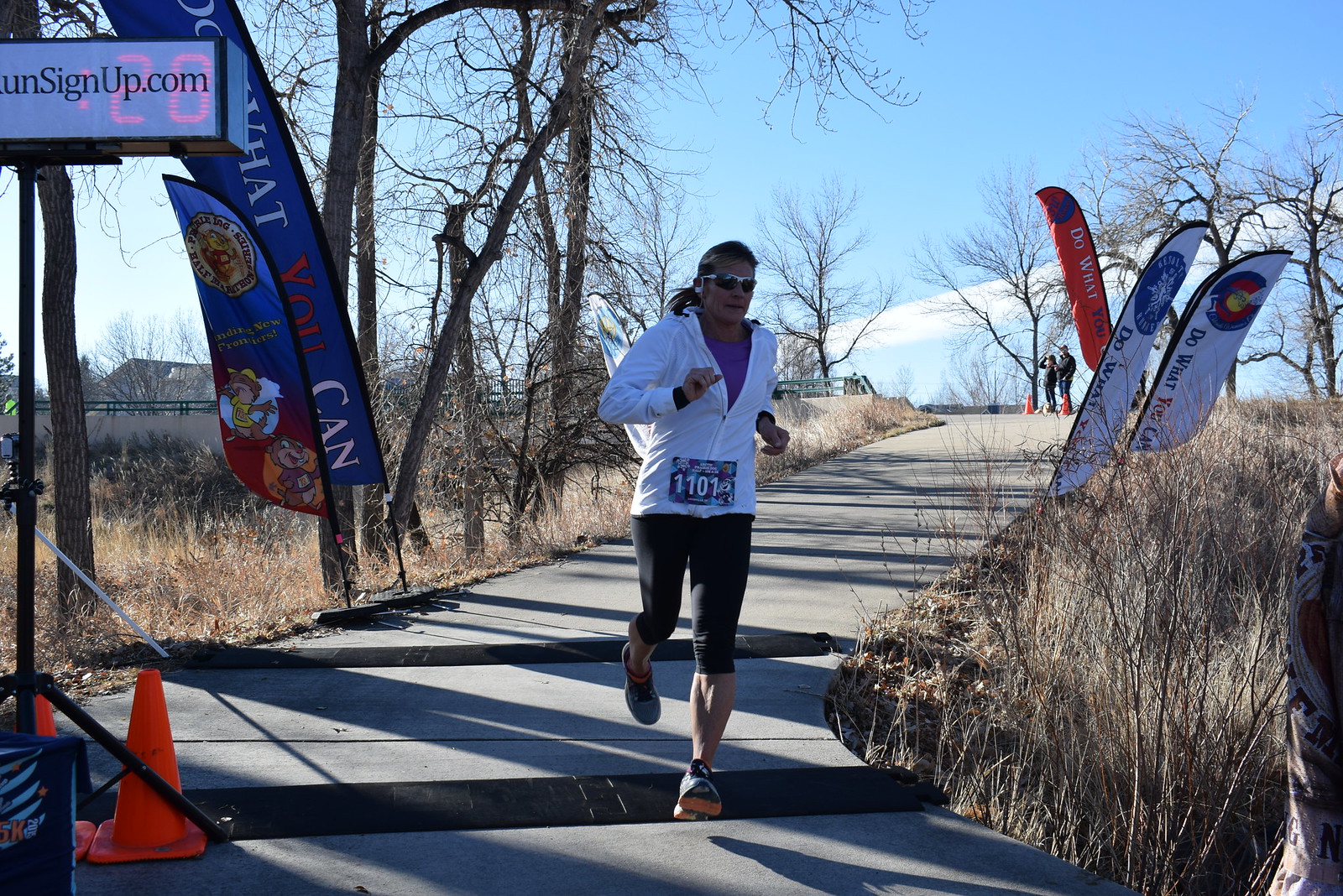In the image, a woman with long brown hair is captured mid-stride, running down a slightly curved, paved path. She is participating in a race, evidenced by the number bib pinned to her white, zip-up jacket. Beneath the jacket, she wears a purple top, paired with black knee-length leggings and running sneakers. The front of her body is in shadow, suggesting a backlit setting.

The path is flanked by several tall, feather-like banners, some of which feature inspirational messages like "do what you can," while others display cartoon graphics. Cones and signs are set up along the track, guiding participants. Two signs on her right and three on her left, colored white, red, and blue, add to the structured race environment. 

In the background, a few spectators stand on either side of the path, watching the lone runner. The surroundings include brownish winter grass and leafless trees, indicating a cold season despite the bright blue sky with scattered white clouds. A digital timer displaying "28" is positioned above the path's end, tracking the runner's progress as she makes her way towards what might be the finish line.